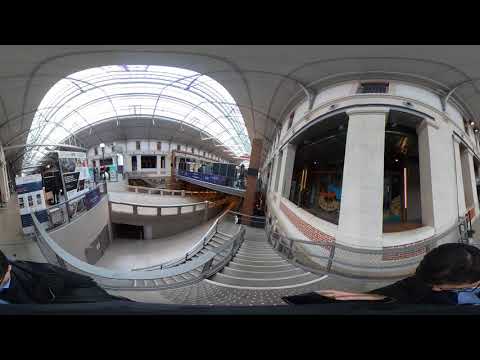The image depicts an expansive indoor scene, resembling a shopping mall, taken with a 360-degree camera. Dominating the structure are two large, eye-like circular formations, one on the left and one on the right, each anchoring their sides of the space. These circles are linked by silver poles and delineated by white pillars. The right circle features prominent stone-white columns, while the left incorporates a bridge-like walkway. Descending into the foreground of the image, a metal stairwell splits into levels, with steps leading to a lower platform and then further down to the floor below. Additional angled ramps and walkways flank the stairwell on the left. The environment is brightly illuminated by a windowed glass roof, allowing natural light to cascade through the structure. The backdrop includes dark spaces and shopfronts, maintaining a stark contrast to the glowing center. People are scattered near the bottom of the image, heads bowed and identities obscured.